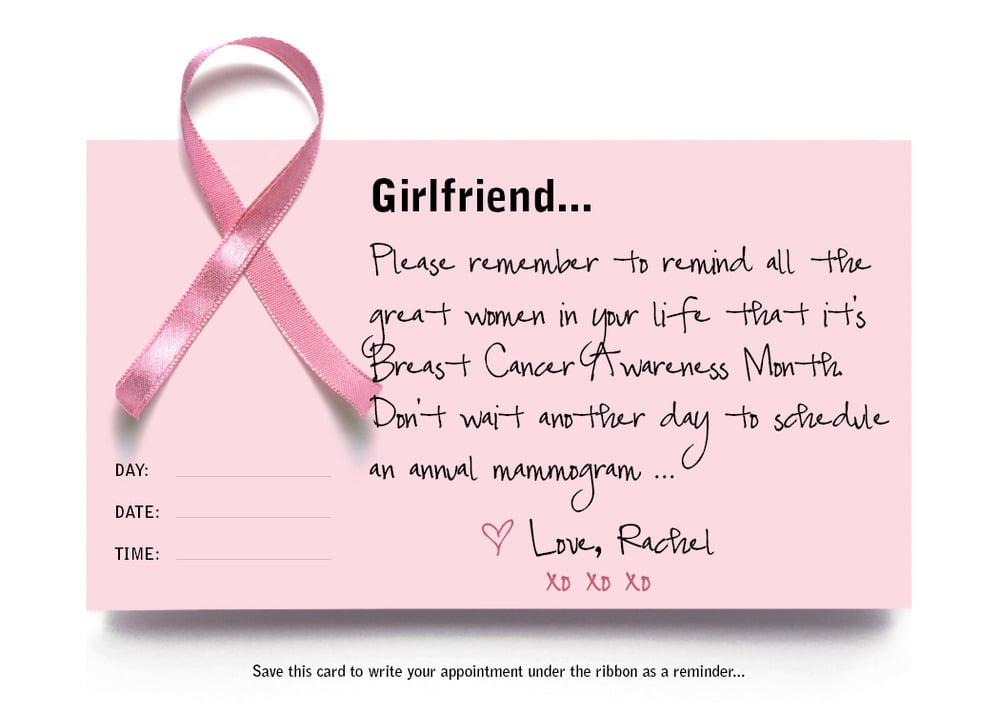The image depicts a rectangular breast cancer awareness card with a soft light pink background. At the top left corner, a realistic pink ribbon illustrates the symbol for breast cancer awareness. The card's bold black heading reads "Girlfriend..." followed by a handwritten-style script that says, "Please remember to remind all the great women in your life that it's breast cancer awareness month. Don't wait another day to schedule an annual mammogram." Below this message, a small pink heart is accompanied by the text "Love, Rachel" and pink "XOXOXO." Towards the bottom, there is a designated area under the ribbon for writing appointment details, labeled "Day," "Date," and "Time" with blank lines to fill in. The card also includes an instruction in small black text at the very bottom: "Save this card to write your appointment under the ribbon as a reminder."